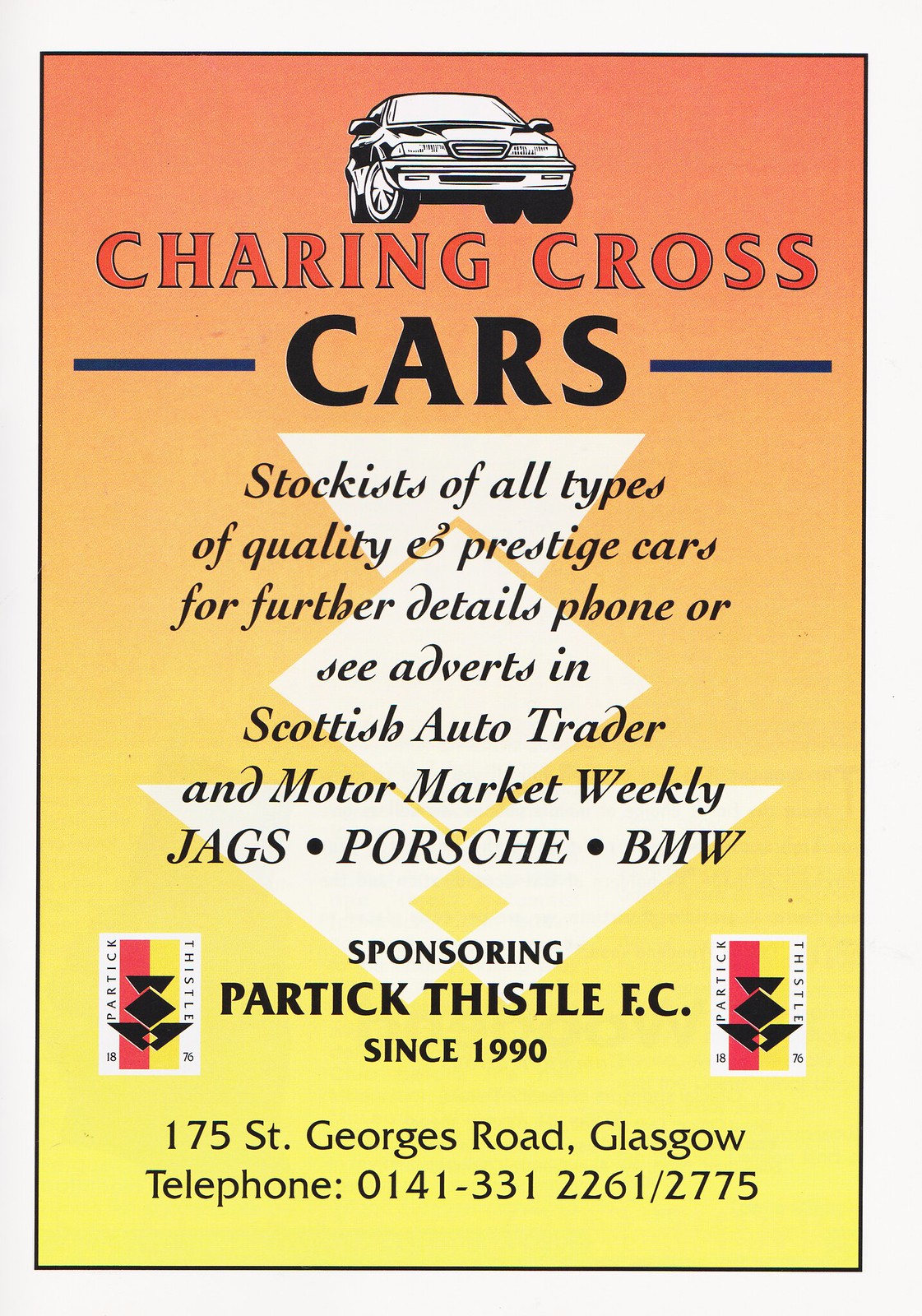This vibrant color advertisement for Charing Cross Cars features an eye-catching background that transitions from orange at the top to yellow at the bottom. Dominating the top of the image is a black and white clipart image of a vehicle. Below this, in large red letters, it says "Charing Cross," with "Cars" prominently displayed in black. 

The ad details the dealership's offerings, stating, "Stockists of all types of quality and prestige cars." It invites potential customers to "phone or see adverts in Scottish Auto Trader and Motor Market Weekly" for more details. Notable brands like Jaguars, Porsches, and BMWs are highlighted. 

Further down, the advertisement proudly notes that Charing Cross Cars has been "Sponsoring Partick Thistle F.C. since 1990." The dealership's address is listed as "175 St. George's Road, Glasgow," along with the telephone number "0141-331-2261/2775." 

Subtle design elements such as blue lines on either side of the word "Cars," and possibly some flags featuring "Partick Thistle" add to the overall detailed composition of the ad.